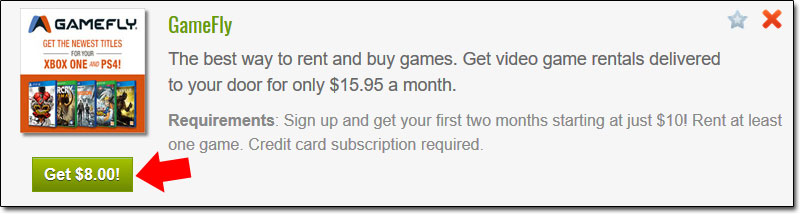This is a detailed screenshot from the Gamefly website. The image is rectangular, approximately four times wider than it is tall, featuring a light bluish-gray background. In the top left corner, there is a small square, about two inches by two inches, split horizontally. The top half of the square has a white background showcasing a stylized Xbox controller graphic. The controller is blue on the left side, black in the center, and red on the right side. Below this, the word "Gamefly" is written in black, and beneath that, in red text, are the words "Get the newest titles 4U." Flanking the text "4U" are two black lines. Further down, in bold red letters, it says "Xbox One and PS4!"

The bottom half of the square has an orange background with five blurry images of video games in the following color-bordered sequence: blue, green, blue, green, and blue.

To the right of the square, there is a prominent green tab that says "Get $8" in white text, accompanied by a thick arrow pointing towards it. Adjacent to the tab, the words "Gamefly" are displayed in green. To the right of this, there is a red 'X' and to its left, a small light blue star.

Below this section, the text "Gamefly" reappears, followed by the tagline "The best way to rent and buy games." Below the tagline, it states, "Get video game rentals delivered to your door for only $15.95 a month."

Further down, there is a smaller section of text detailing the requirements: "Sign up and get your first two months starting at just $10! Rent at least one game. Credit card subscription required."